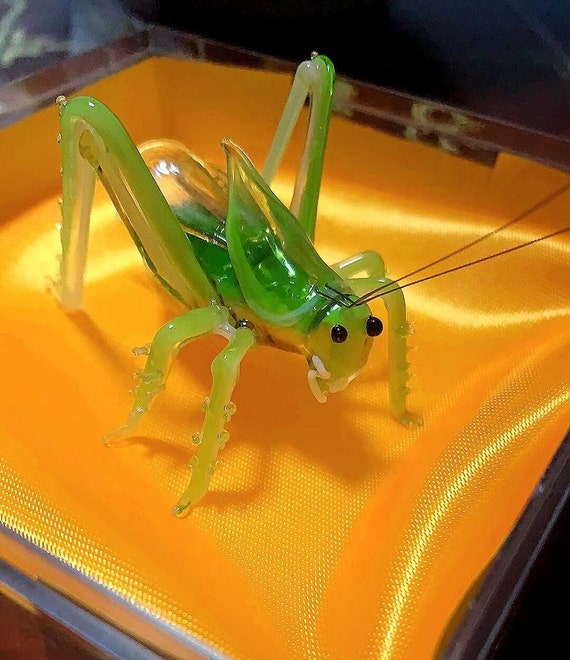This photograph is a detailed close-up, possibly a lab project, featuring an intricately designed artificial grasshopper. The grasshopper is crafted from a shiny, glossy material, likely glass, and showcases a vibrant green hue. It has distinct, large black eyes and delicate antennas resembling thin strings. Its legs are highly detailed, with the back legs propped up as if in a crouching pose. The insect's body is textured and appears to have a slightly slimy sheen, enhancing its lifelike appearance.

The grasshopper is set atop a slightly porous, shiny orange fabric or platform, which could be a decorative bowl or plate. The bright, golden yellow color of the fabric contrasts vividly with the green of the grasshopper, making the colors in the image pop. The perspective of the photograph is very close, capturing the fine details and textures, and overall, the image quality is high. There are no texts present in the image.